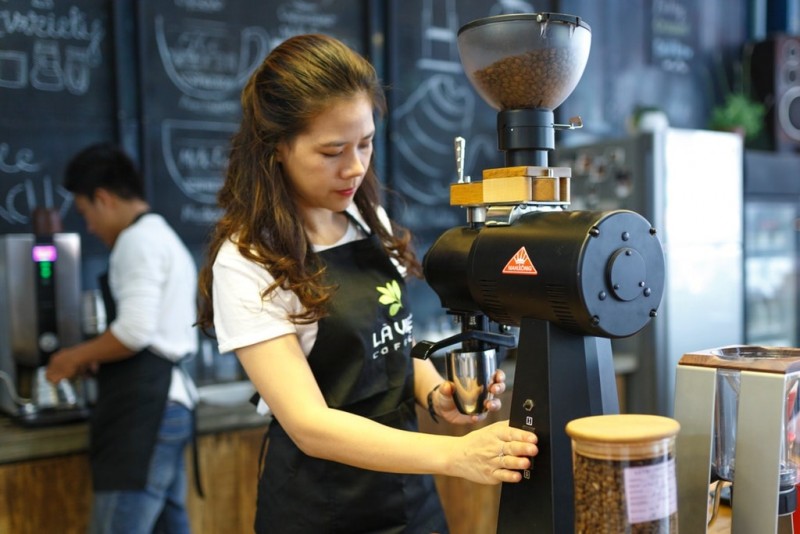In this vibrant scene inside a bustling coffee shop, two baristas work diligently behind the counter. Dominating the right foreground, a woman with long brown hair, possibly of Asian descent, wears a white T-shirt and a black apron emblazoned with "Lave Coffee." She is focused on operating a large, black coffee machine. With her right hand, she presses a button or lever on the machine, which features a bowl of coffee beans at the top with a wooden design. Coffee pours into a silver cup held in her left hand. On the counter in front of her, additional containers of coffee beans are visible. To her right, in the background, a male coworker is also engaged in preparing coffee. He sports a white shirt, blue jeans, and a black apron, his short brown hair neatly styled. Behind them, black chalkboard frames hang on the walls, adorned with various chalk drawings and menu information. A speaker sits atop one of the adjacent cases, contributing to the lively ambiance of the shop.